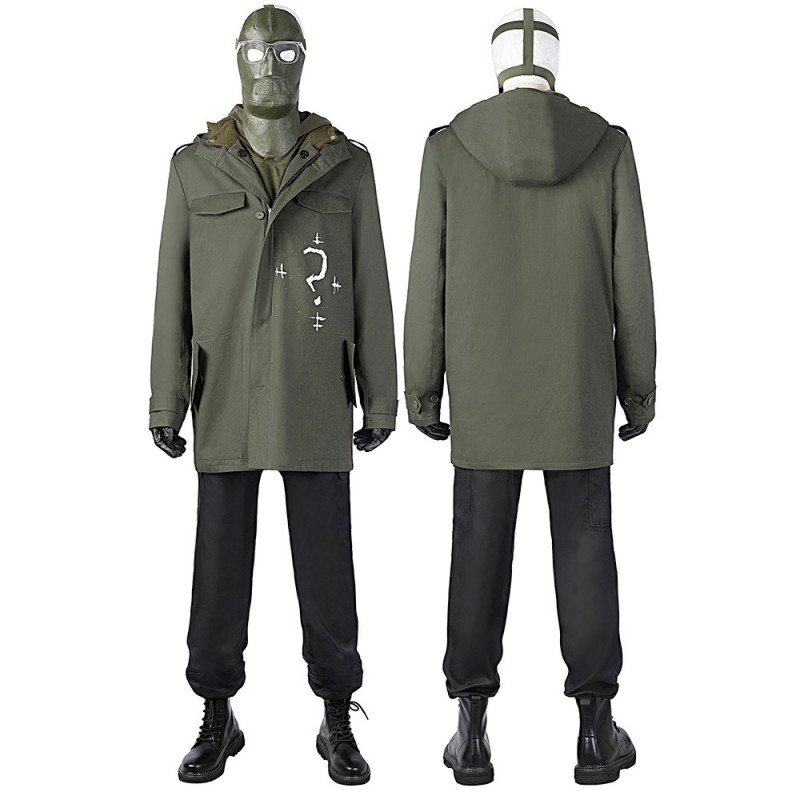This photograph showcases a meticulously detailed costume inspired by the Riddler from the 2022 film "Batman." The outfit features shiny black lace-up boots paired with black pants, creating a sleek, ominous look. Over these, the wearer dons a large green army jacket with an attached hood and black leather gloves. The jacket’s left side (our right) is emblazoned with a white question mark, surrounded by four unique crosses, each with two strikes through them, positioned at the cardinal points.

The upper part of the costume includes a full facial mask that completely covers the person's head and neck, with only eye cutouts and small mouth holes for breathing. The mask is a grayish-green hue, topped with clear glasses. An olive green t-shirt is visible beneath the jacket, adding another layer of detail.

The photograph also provides a rear view of the ensemble, revealing that the jacket has a hood and the mask is secured with visible straps. The back of the coat is plain, emphasizing the utilitarian design of the outfit. Overall, the costume is a faithfully eerie representation of the Riddler's attire, capturing the character's menacing and enigmatic presence.